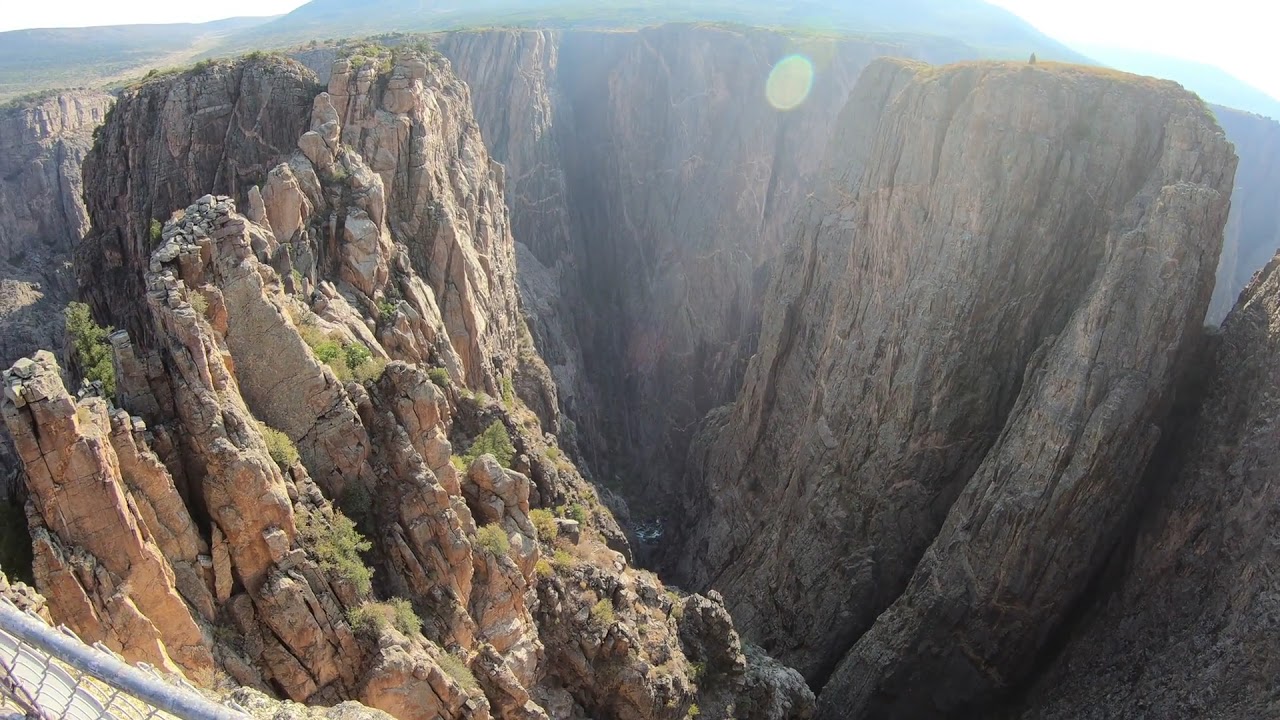This photograph captures a scenic vista looking down into a vast, jagged canyon or gorge with rugged, mountainous ridges. Dominating the foreground, on the bottom left, is the top edge of a chain-link fence, indicating a vantage point designed for safety. The rocky cliffs, displaying hues of limestone, orange, brown, burnt orange, green, and beige, carve out dramatic, steep slopes that plummet into shadowy depths obscured from view. On the left side, a significant canyon divides the landscape with a zigzag pattern, while a massive dip on the right contrasts starkly with a jutting cliff that rises sharply, crowned by sparse grass and a solitary tree. The bright, sunny day adds a slight haze to the scene, casting parts of the canyon into shadow. In the distance, more cliff formations stretch out, appearing white and blue under the clear horizon dotted with white clouds. The entire setting is suffused with natural light, enhancing the vibrant, multi-colored texture of the rocky terrain.